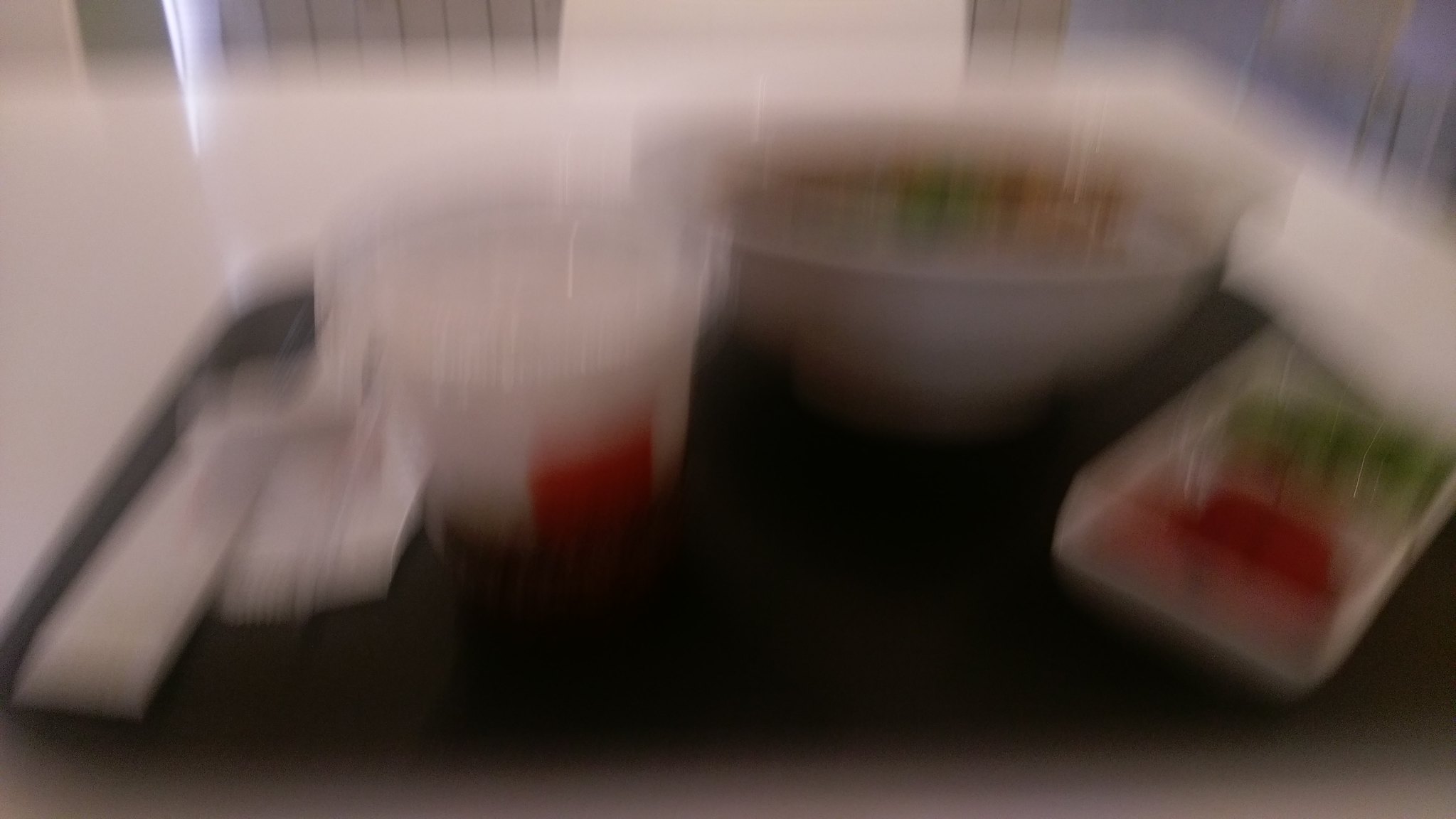This image is notably blurry, capturing a scene set on what appears to be a black or brown tabletop. The table features an assortment of containers:

1. **Gray Bowl**: Contains a mixture of green and brown, possibly food items.
2. **Round Container**: Either clear or white, adorned with a distinctive red strip.
3. **Rectangular Container**: Transparent and divided into sections; one section holds a red substance, and another contains green.

In addition, there is a nondescript white item on the table. Surrounding the table is a blurred white area. The background is more discernible, showing a wall or surface with white elements transitioning into green. Further details reveal gray vertical panels divided by a white strip, then additional gray panels. In one corner, a bluish-purplish-gray blur can be observed.